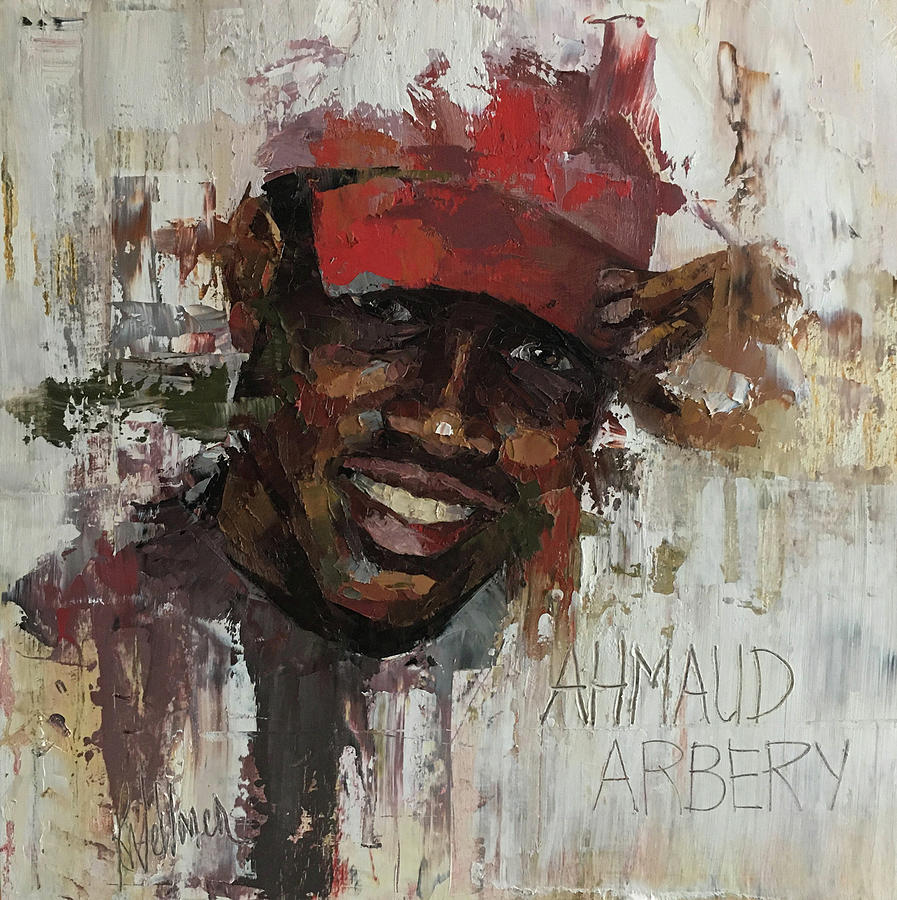This abstract painting, styled with a technique that uses varying paint textures and intensities, portrays Ahmaud Arbery, a black man who was sadly killed. The subject, who appears to be between 20 and 40 years old, is depicted with dark skin and a radiant smile that reveals his teeth and shiny eyes. He is wearing a red baseball cap and is shown with his hand touching or adjusting the bill of the cap. The background features a blend of gray, white, beige, and other subtle hues, providing a contrasting backdrop to the vivid figure. In the bottom right corner, the name "Ahmaud Arbery" is inscribed, possibly in brown paint or ink. There is also an illegible signature on the bottom left, indicating the artist’s mark. The painting's style, somewhat resembling a smear or scraped technique, lends a dynamic and textured feel, bringing Ahmaud’s likeness to life in a manner that appears both true to him and emotionally evocative.